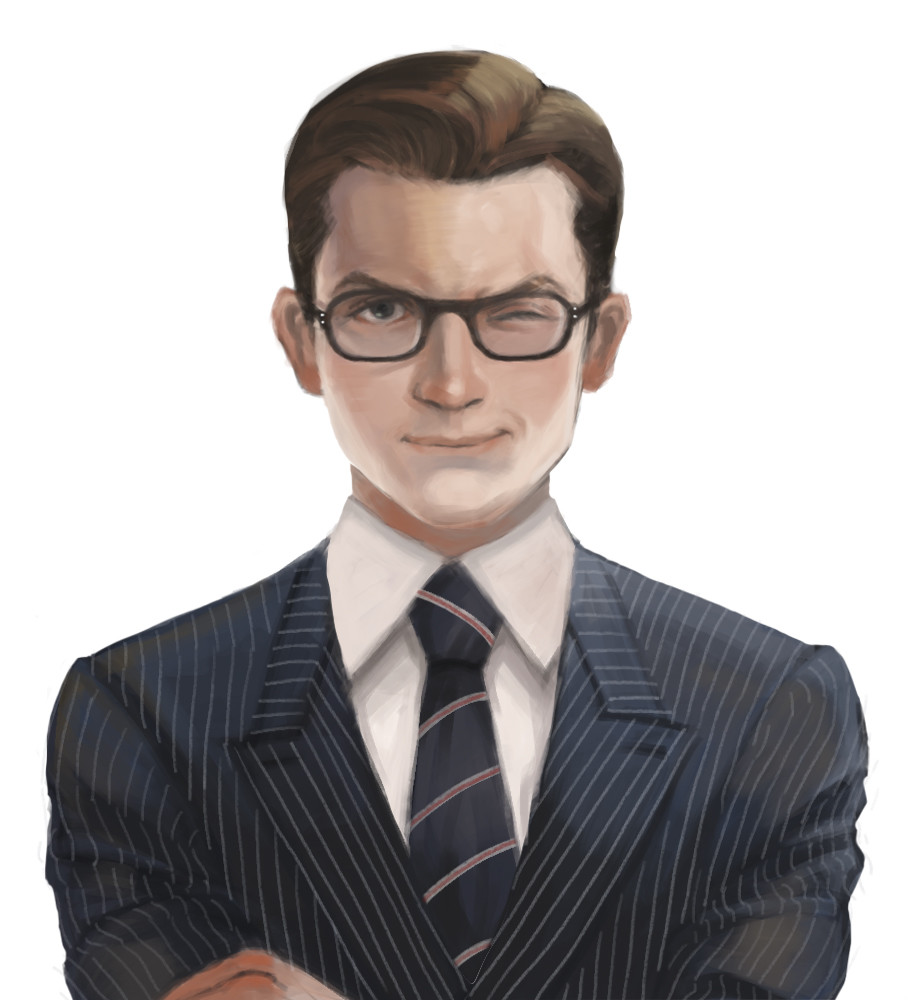This is a detailed illustration of a sharp-looking man appearing to be in his late 20s, depicted from the waist up. His brown hair is neatly parted on the left and combed over, cut short around the sides and ears. He wears dark brown or black rectangular glasses, with a slight roundness to the edges. His expression is characterized by a playful smirk, with one eye winking on the left side of the image. His eyebrows are brown, and his visible eye appears to be gray.

He's dressed in a tailored pinstripe suit, black with thin white stripes running vertically. Underneath, he sports a crisp white collared button-down shirt, and a tie that is either navy blue or black, decorated with diagonal red and gray stripes. His arms are folded in front of him, with only part of his knuckles visible on the lower left side of the image. The overall composition, style, and detailed elements suggest that this image is either a sketch or a painting.